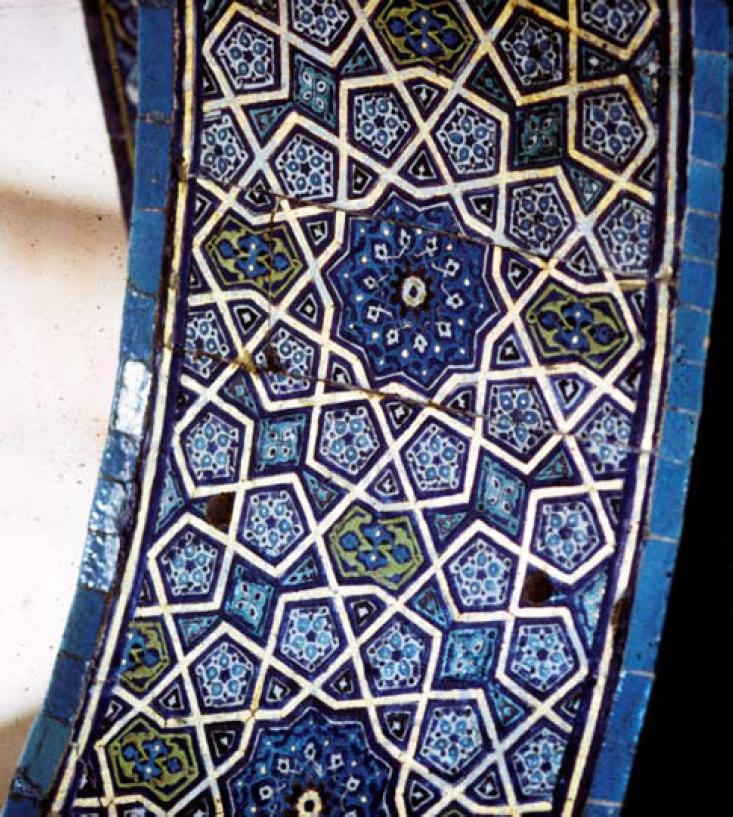This close-up photo captures the intricate details of a blue-toned ceramic mosaic tile, possibly part of a larger display. The tile features a prominent, dark blue nine-sided star with a white center at its core, surrounded by an array of lighter blues, baby blue, and touches of indigo. Interwoven with these shades are accents of pale olive green, contributing to a vibrant, colorful palette. The tile's design is complex and geometric, with patterns forming a flowery effect that is highlighted by a white zigzag border interspersed among the other elements. There are visible cracks on the tile, hinting at its age and adding to its character. The background to the right of the tile is black, emphasizing the tile's curvature and serving as a subtle frame for the piece. Although the exact location and original purpose of the tile are unknown, its elaborate design and signs of wear suggest it might be an ornamental piece on display.